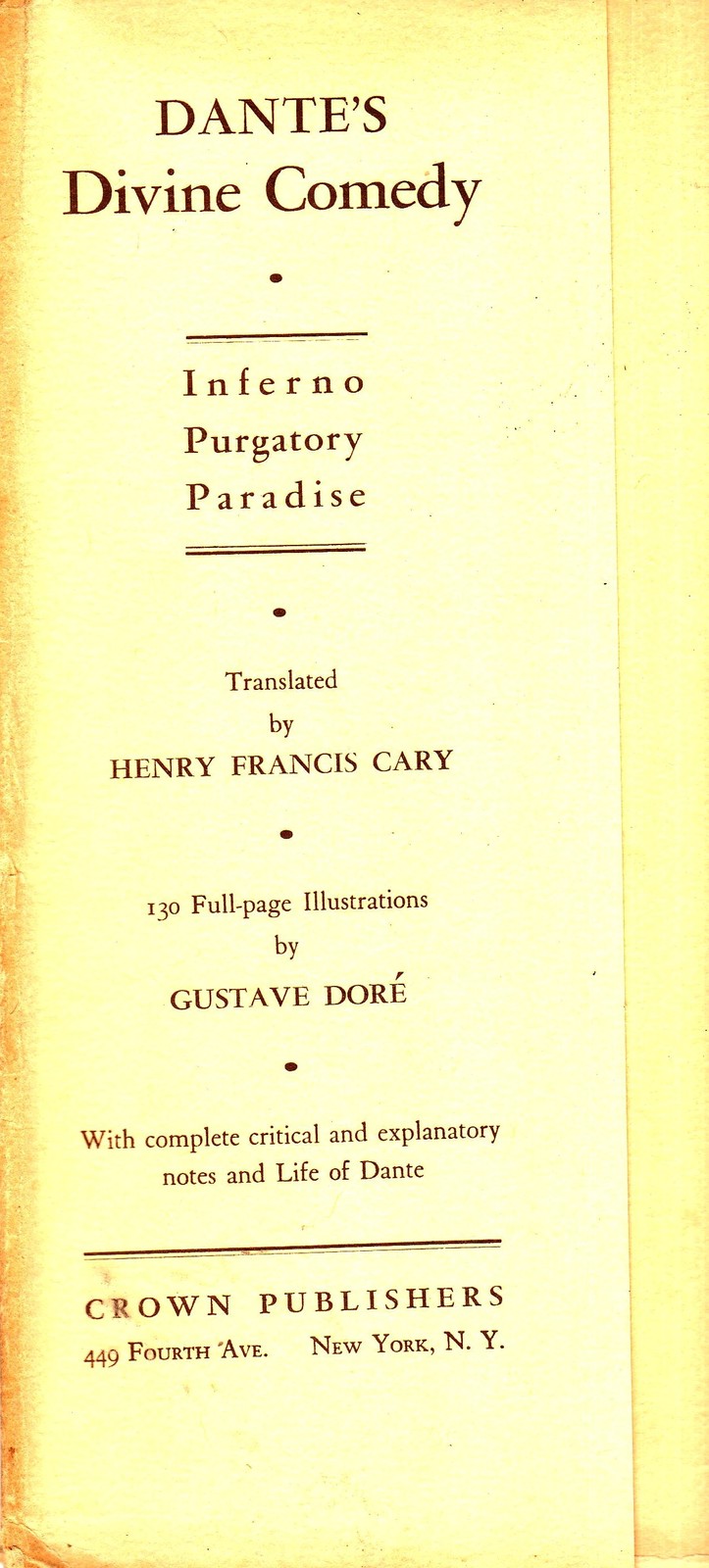This image features a vintage, off-white or eggshell-colored first page of a book, framed within a tall vertical rectangle. At the top, the title reads "Dante's Divine Comedy" in black text, followed by a dot beneath it. A horizontal line is situated below the dot, and underneath this line, three lines of text read "Inferno," "Purgatory," and "Paradise." Another horizontal line appears after this trilogy, followed by two horizontal lines beneath it. A dot marks the next section, followed by the text "Translated by" in capitalized font, with "Henry Francis Carey" written below. Another dot follows, then the text "130 full-page illustrations" with the numbers in numerals, attributed to "Gustave Doré" in uppercase letters. A subsequent dot leads to the text "With complete critical and explanatory notes," with the following line mentioning "Life of Dante." Two final horizontal lines, with the top one thicker, frame the lower section where "Crown Publishers" is written in uppercase letters. At the bottom left, the address "449 4th Ave.," and on the bottom right, "New York, N.Y." is stated. The page exhibits a yellowish or sepia-toned hue, indicating its vintage nature.